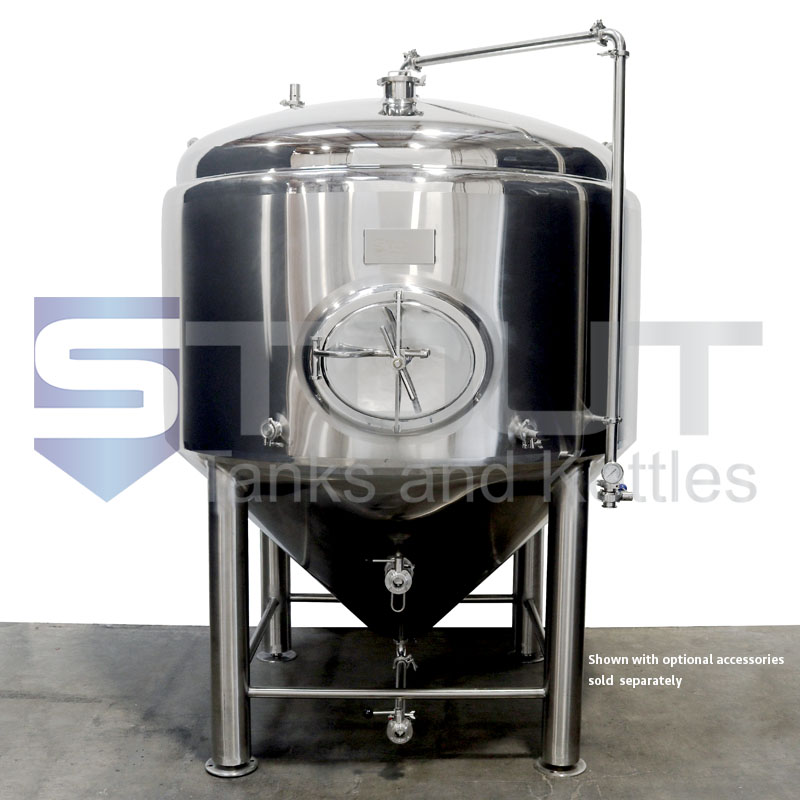This color photograph showcases a brand-new, large still intended for brewing liquids such as beer or kombucha. The image is rectangular, with equal length and size on all sides. The primary focus is a cylindrical stainless steel container featuring a conical bottom that tapers towards a valve and pipe. The tank is securely set into a metal frame with cylindrical legs. At the very top, a metal tube extends from the still, running along the side and equipped with a valve and gauge on the right. A notable feature is the central circular doorway, which includes a large rod mechanism for locking.

Overlaying this image is semi-transparent text that reads "stout" or "stilt tanks and kettles," although the exact brand name is difficult to discern due to the gray letters blending into the shiny silver background. Additionally, small text at the bottom right of the photograph states "shown with optional accessories sold separately." The overall presentation lacks color contrast, making the text hard to read against the reflective surface of the new stainless steel tank.